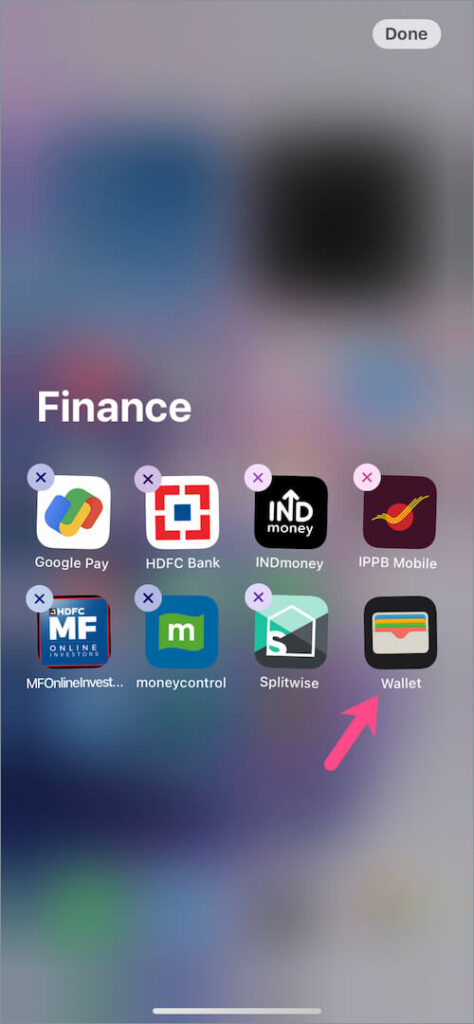This screenshot captures the home page of a device, specifically showcasing a folder titled "Finance" in white text on the left side of the screen. The folder contains eight app icons, neatly arranged in a grid of four icons per row.

In the first row, the icons are as follows:
1. **Google Pay** - Represented by a colorful money sign in the four signature colors of the Google logo: blue, green, yellow, and red.
2. **HDFC Bank**.
3. **IndMoney**.
4. **IPPB Mobile**.

In the second row, the icons are listed as:
1. **MF**.
2. **Online Invest**.
3. **Money Control**.
4. **Splitwise**.

The final icon in the second row is labeled **Wallet** and is distinguished by a red arrow pointing diagonally upward to the right.

At the top of the screen, a pill-shaped white button is present, labeled "Done". Additionally, small purple X's are visible next to the first seven app icons, suggesting that they can be removed or edited.

The overall layout and arrangement convey a user's organized approach to managing their financial applications in one accessible location.